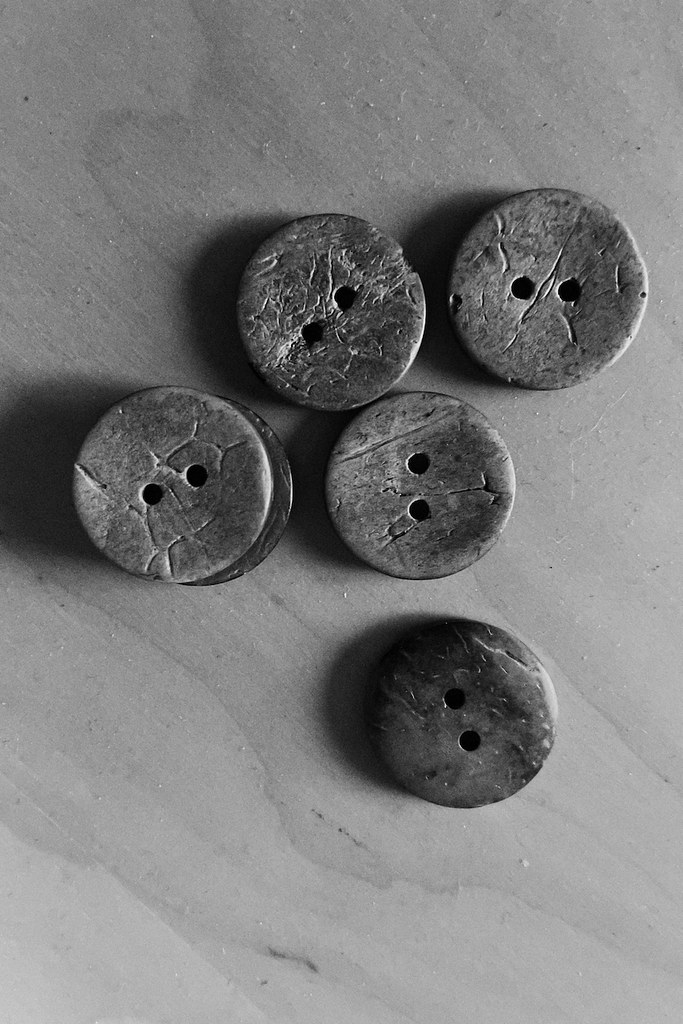This black-and-white photograph captures six worn, round, wooden buttons arranged on a light wood surface, possibly pine. Each button features two centrally aligned holes and displays distinctive scratch marks and crevices, suggesting age and use. The buttons range in color from slightly dark to lighter gray hues. An interesting arrangement shows two buttons stacked with one lighter button on top of a darker one, while the remaining four are laid out individually. Positioned in a unique formation, three buttons align horizontally with two extending downward, somewhat reminiscent of a snowman with outstretched arms. The surface beneath the buttons displays visible wood grain, adding texture to the image, and the lighting casts subtle shadows to the left of each button.